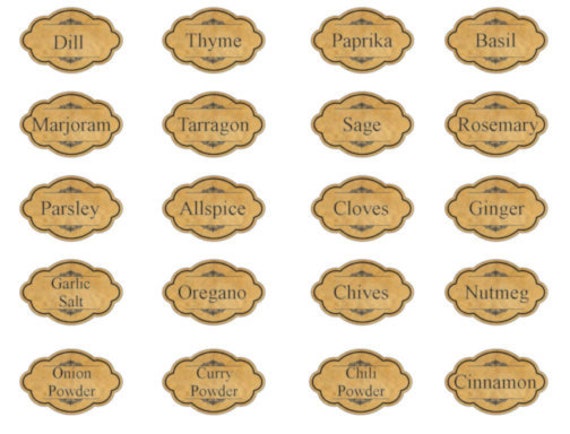The image depicts an organized array of 20 spice labels, set against a white background. The labels are displayed in brown, undulating ovals with black text, orderly arranged into five rows of four spices each. The top row includes dill, thyme, paprika, and basil. The second row features marjoram, tarragon, sage, and rosemary. The third row lists parsley, allspice, cloves, and ginger. Following this, the fourth row shows garlic salt, oregano, chives, and nutmeg. Finally, the bottom row consists of onion powder, curry powder, chili powder, and cinnamon. Each label, highlighted by its yellow and gray tones, distinctly identifies the spice within these uniformly shaped ovals.